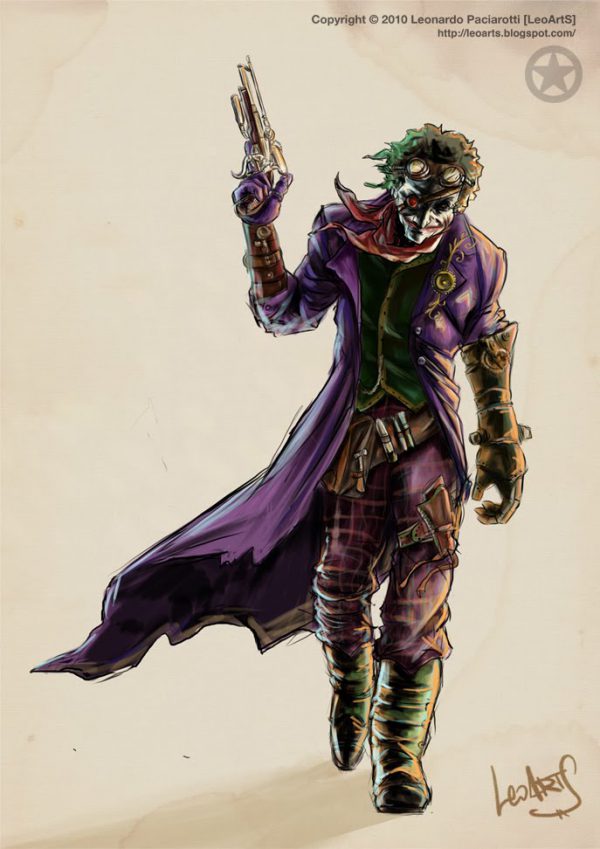This detailed artistic rendering depicts the Joker from Batman, showcasing his iconic look with some unique steampunk elements. He is instantly recognizable by his ghostly white face paint, vibrant green hair, and an exaggerated red mouth. His piercing red eye adds to his menacing appearance, and a red scarf elegantly drapes around his neck.

The Joker is dressed in a long, flowing purple trench coat and matching purple pants. He sports a green vest underneath, cinched with a brown belt adorned with bullets, and a gun holster strapped to his front left leg. His feet are clad in knee-high black boots, giving him a formidable stance.

His accessories are particularly striking: he wears large, metal gloves that extend up to his elbows, with a steampunk twist featuring copper hues. Goggles rest atop his head, ready to shield his eyes at a moment's notice. In his left hand, he brandishes a golden gun, held confidently aloft.

The background is a simple tan, allowing the intricate details of his costume and accessories to stand out. The top left corner of the image is inscribed with "Copyright 2010, Leonard Panschiart, Leo Art S," followed by the URL "http://leoart.blogspot.com." Below this is a grey circle with a star inside it. The bottom left corner bears the artist's signature, adding an authentic touch to this vivid portrayal of the Joker.